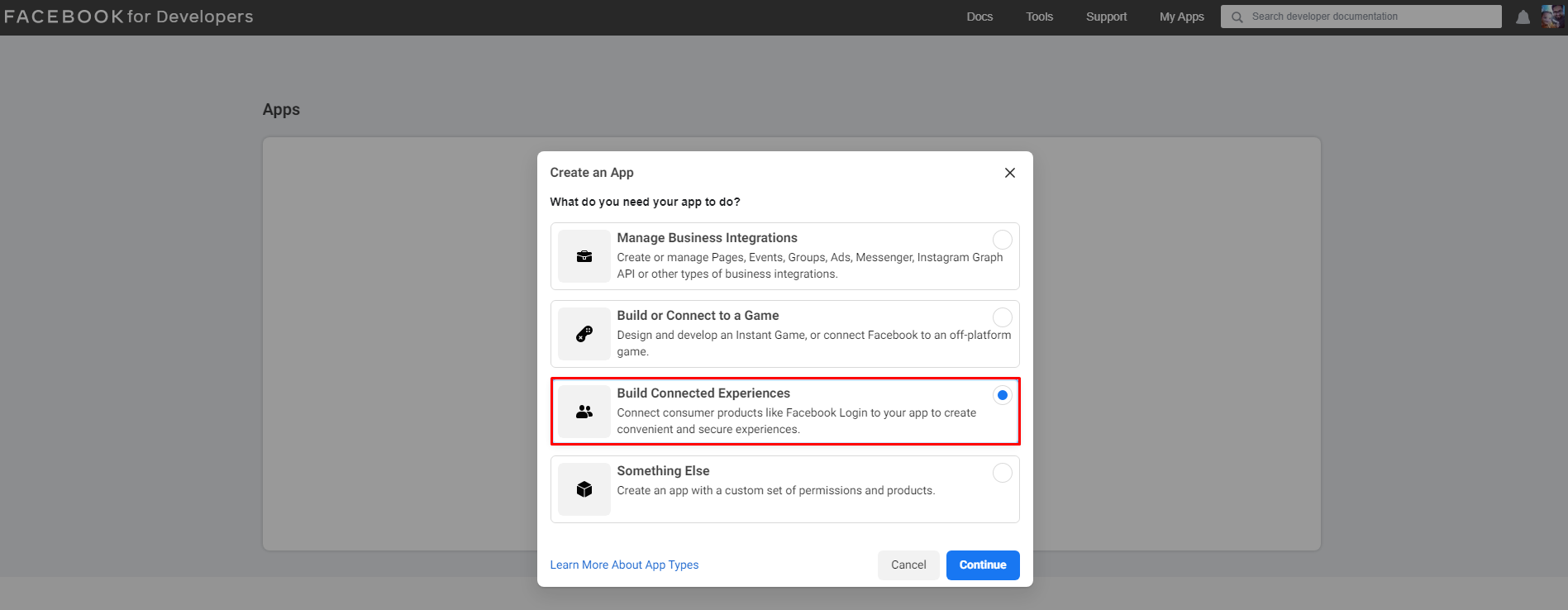**Detailed Caption:**

A screen capture of a pop-up window on the Facebook for Developers page, with the rest of the page dimmed in the background. Central to the image is the pop-up window titled "Create an App." In this window, four rectangular options are displayed, each with a simple black icon to the left:

1. "Manage Business Integrations"
2. "Build for Content"
3. "Build or Connect to a Game"
4. "Build Connected Experiences"

The "Build Connected Experiences" option is outlined in red, highlighting its selection. At the bottom of the pop-up window, there are two buttons: "Cancel" and "Continue" on the lower right, and a link titled "Learn More About App Types" on the left. The highlighted option provides instructions on connecting customer products, such as Facebook Login, to the app for enhanced user experiences, although part of the text is blurry.